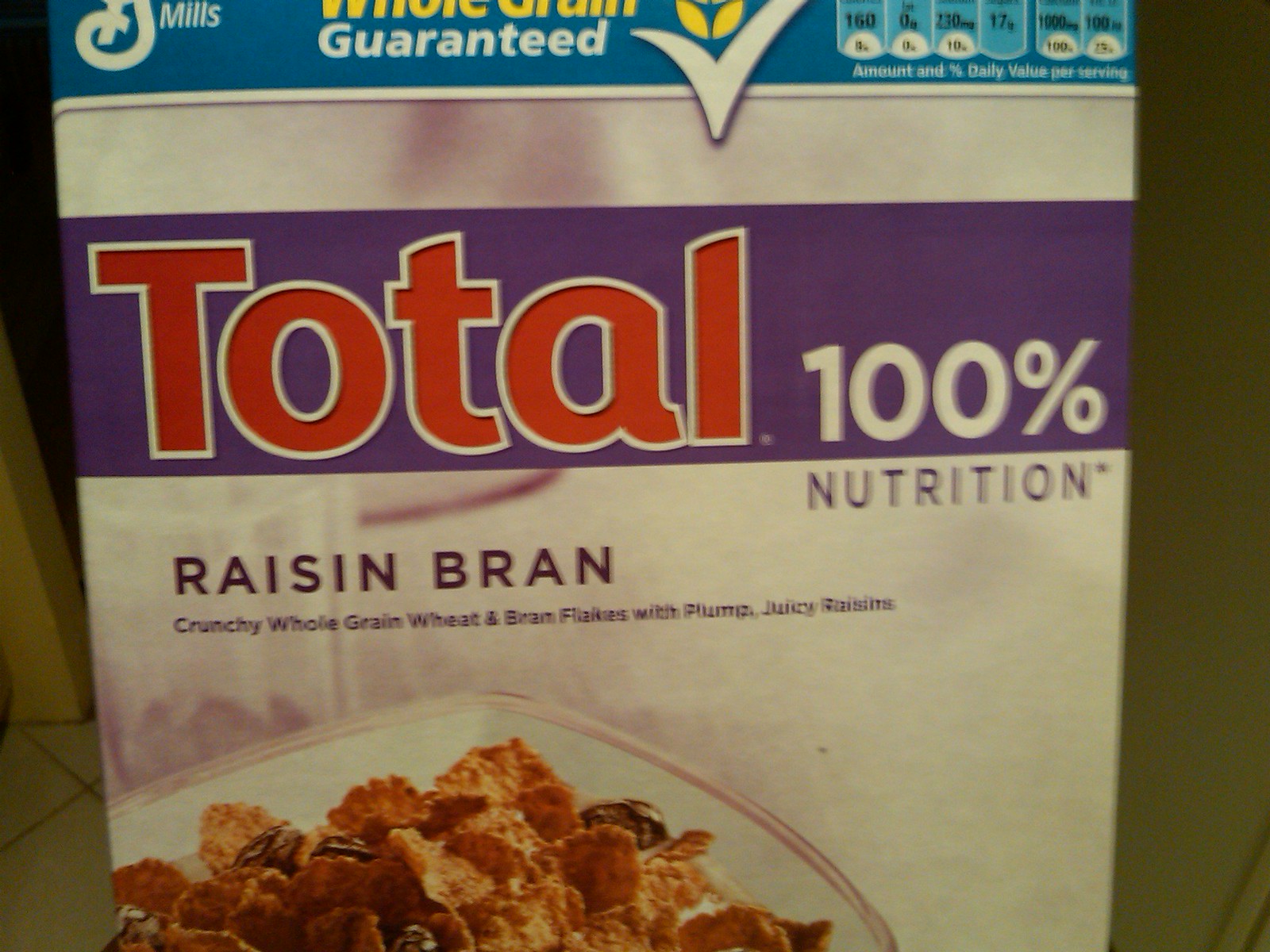The image depicts a slightly wider than tall cereal box of Raisin Bran Total, likely by General Mills. The top part features a blue and purple banner with red text reading "Total" outlined in white, accompanied by white text stating "100% Nutrition" below the banner. Above this, a yellow flower with a white checkmark likely accompanies the phrase "Whole Grain Guaranteed." The partial photograph captures the main branding, but much of the text and logo in the upper portion is cut off, partially showing "Mills" and some daily value percentages like "160", "0", "230", "17g", and "1,000mg." The lower part of the box showcases a bowl of Raisin Bran against a white background with a pink-rimmed, squared-off bowl, filled with crunchy, whole grain wheat, and bran flakes mingled with plump, juicy raisins and milk. To the lower left, there's a glimpse of a grayish tile floor and possibly a yellow door frame corner.